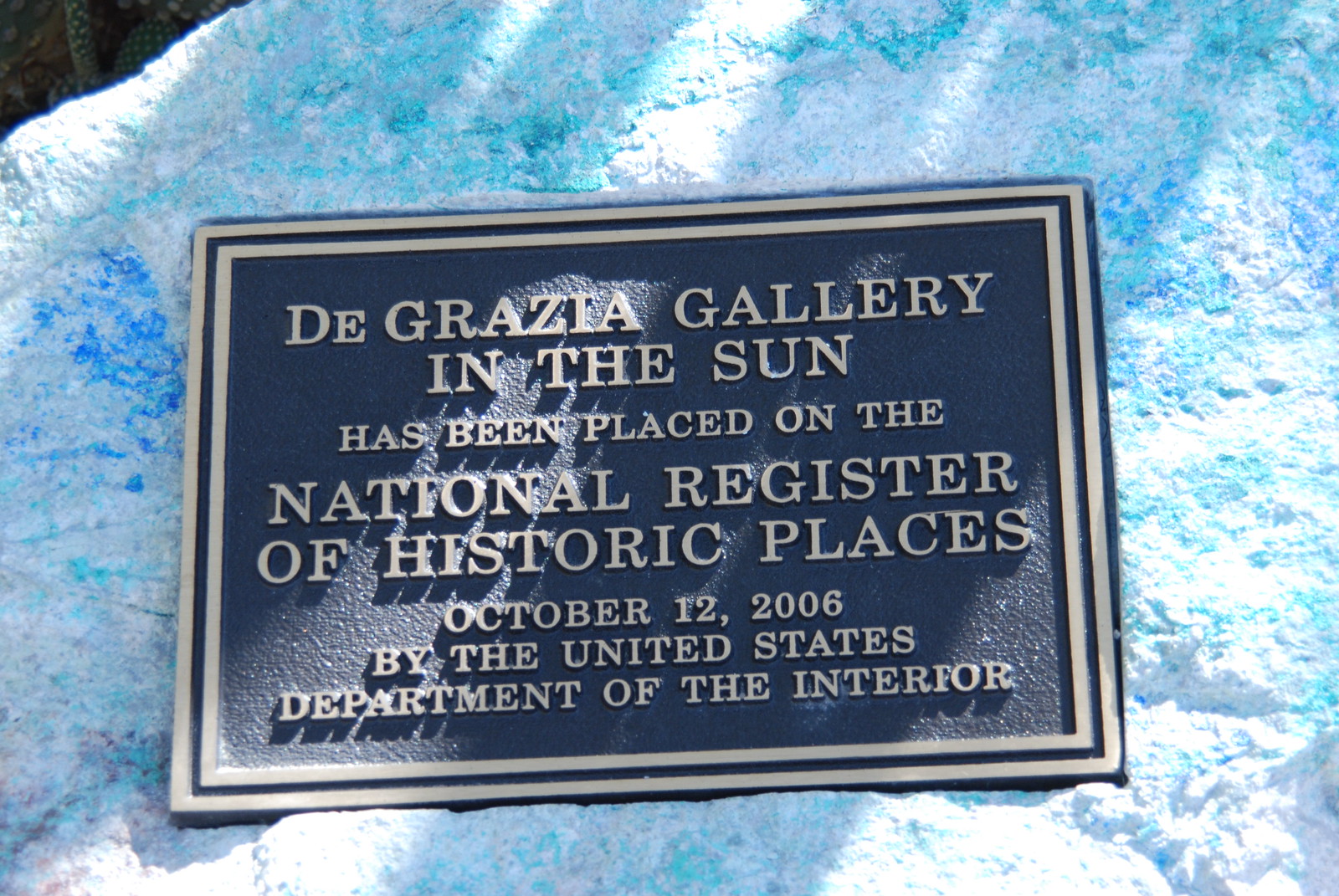The image features a brass plaque with a faded gold inscription against a blackened background, prominently displayed at the center of the frame. The text on the plaque, all in capital letters, reads: "DeGrazia Gallery in the Sun has been placed on the National Register of Historic Places, October 12, 2006, by the United States Department of the Interior." The plaque is mounted on a striking, greenish-blue to turquoise rock formation, which dominates the entire background of the image, with only a small portion of open space visible in the top left corner. The image suggests an outdoor, possibly wooded, setting, and the plaque's surroundings are marked by varied hues of white, light blue, dark blue, and tan, with some shadowing indicating natural light.